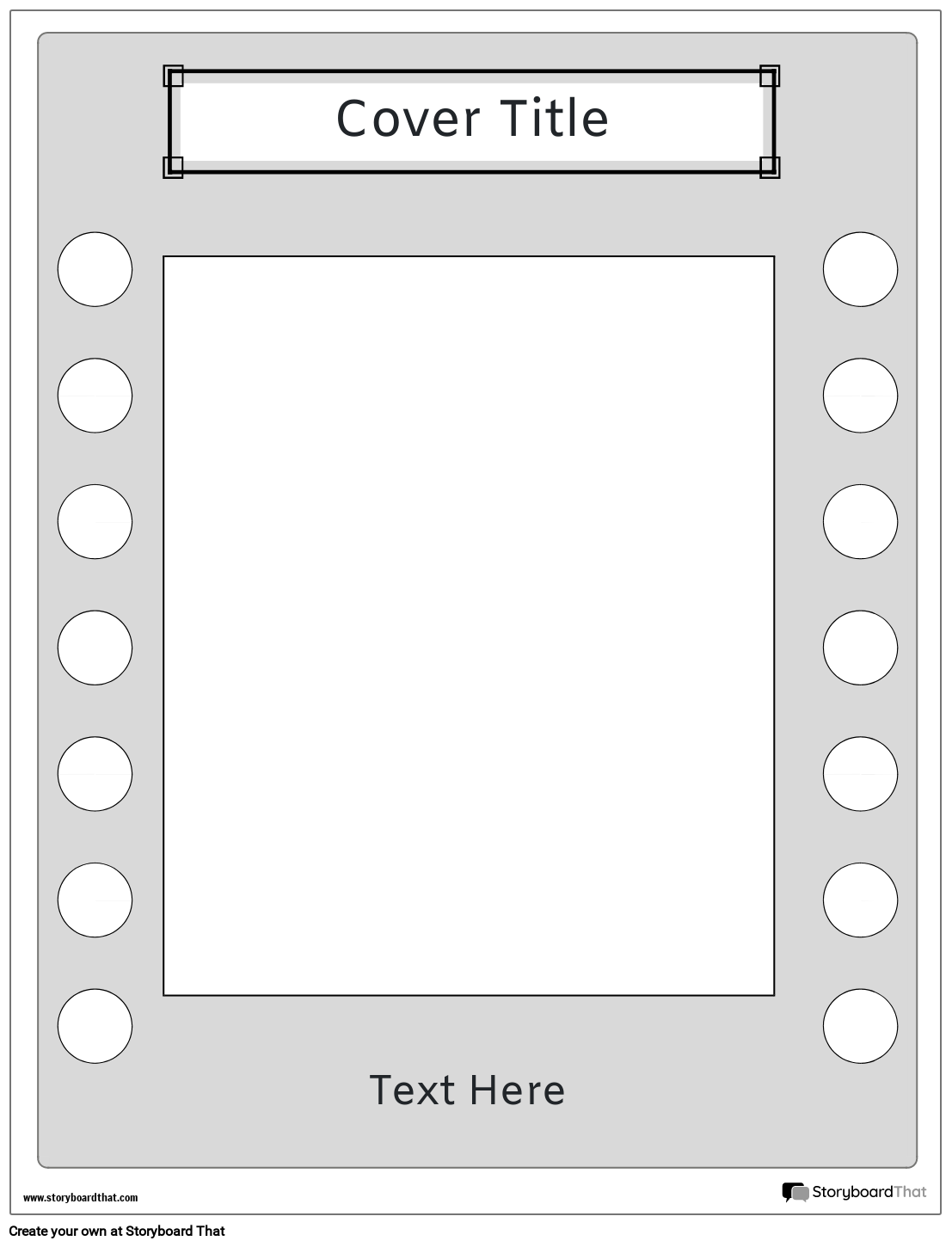The image is a detailed template for a book or report cover, primarily consisting of a line drawing with a light gray frame. The central part of the template is designated for an insert, approximately the size of an 8 by 10 photo, marked by a large blank white space. Above this central area is a rectangle, equally wide, containing the text "cover title" in black letters within a white box. Along the edges of the gray frame, extending vertically from top to bottom, are seven white circles on each side, reminiscent of small spotlights for decorative purposes. At the bottom, there is an additional area for text labeled "text here." Outside the main outline of the template, watermarking from the brand "Storyboard That" is visible. The bottom left corner displays the text "www.storyboardthat.com" and "create your own at storyboard that." Additionally, the logo for "Storyboard That" appears at the very bottom right, reinforcing the branding. This organized layout suggests it is a planning sheet or digital mock-up for someone creating a storybook, report, or other structured document.